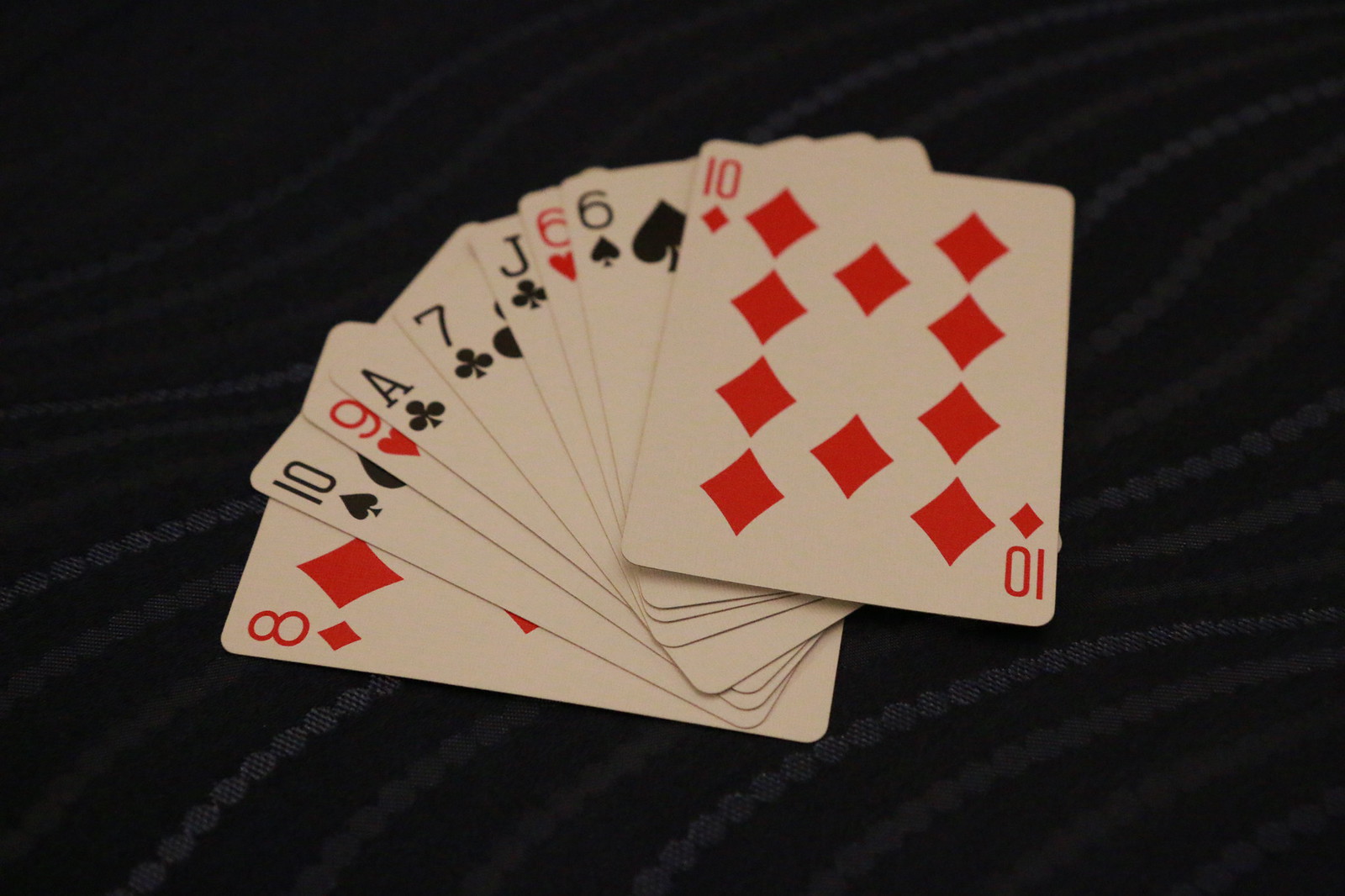The image depicts a black felt card table adorned with an intricate, fine white scroll pattern. Spread out on the table is a nine-card hand, meticulously laid out face-up in the following order from left to right: the Eight of Diamonds, Ten of Spades, Nine of Hearts, Ace of Clubs, Seven of Clubs, Jack of Clubs, Six of Hearts, Six of Spades, and finally, the Ten of Diamonds. The cards seem slightly aged, possessing an antique quality with edges that have dulled to a grayish hue, contrasting the bright, crisp images typically found on newer cards. The arrangement suggests the possibility of crafting a straight, hinting at a game of poker, though no other game elements are visible in the photo. The table's elegant design and the vintage feel of the cards add a touch of sophistication and nostalgia to the scene.